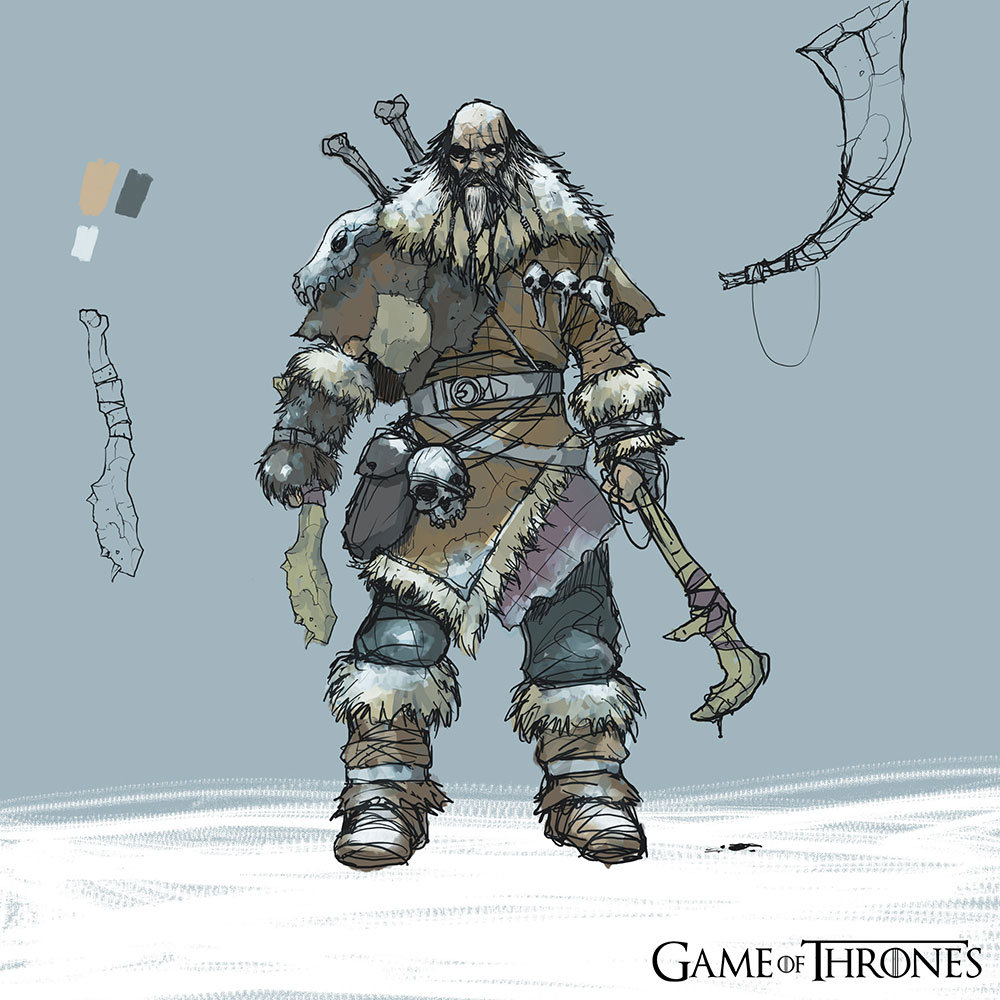The image depicts a hand-drawn character design for "Game of Thrones," as indicated by the title in the bottom right corner. The setting features a grayish-blue background with sketch marks and color palettes on the left. The character is a large, fierce-looking man, possibly a wildling, with a bald head on top, black hair on the sides, and a thick black and gray beard. He is clad in a heavy brown winter coat trimmed with white fur. 

Various skulls adorn his figure: a large animal skull rests on his left shoulder, smaller skulls serve as jewelry on his chest, and a human skull is tied around his waist. He is armed with multiple weapons; bone-like weapons protrude from his back and in each hand, he holds a different implement: a knife in his left and a bone club in his right. His appearance suggests he is braving a snowy environment, prepared for battle.